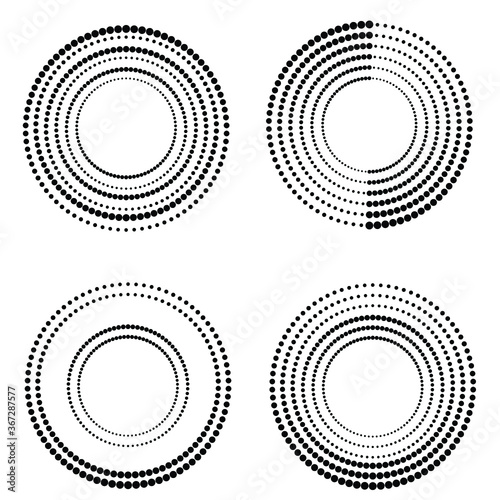The image features four distinct circular patterns arranged in a 2x2 grid, each formed by varying sizes of black and white dots that transition from dark to light. The circles appear uniform in size but differ in the number and arrangement of dot rings. Each circle has a white center and white spaces in between the dots. The top left circle is composed of six concentric rings, with dot sizes fluctuating from larger to smaller in a specific sequence. The top right circle also contains six rings, with dots shrinking uniformly towards the center. The bottom left circle consists of four rings; two inner rings are tightly packed, while the two outer rings are more spaced out, creating a pronounced gap in the middle. The bottom right circle returns to a six-ring structure, with the inner three rings featuring larger dots and the outer rings showcasing a reverse pattern. The text "Adobe Stock" with the identifier "367287577" appears along the left side of the image.